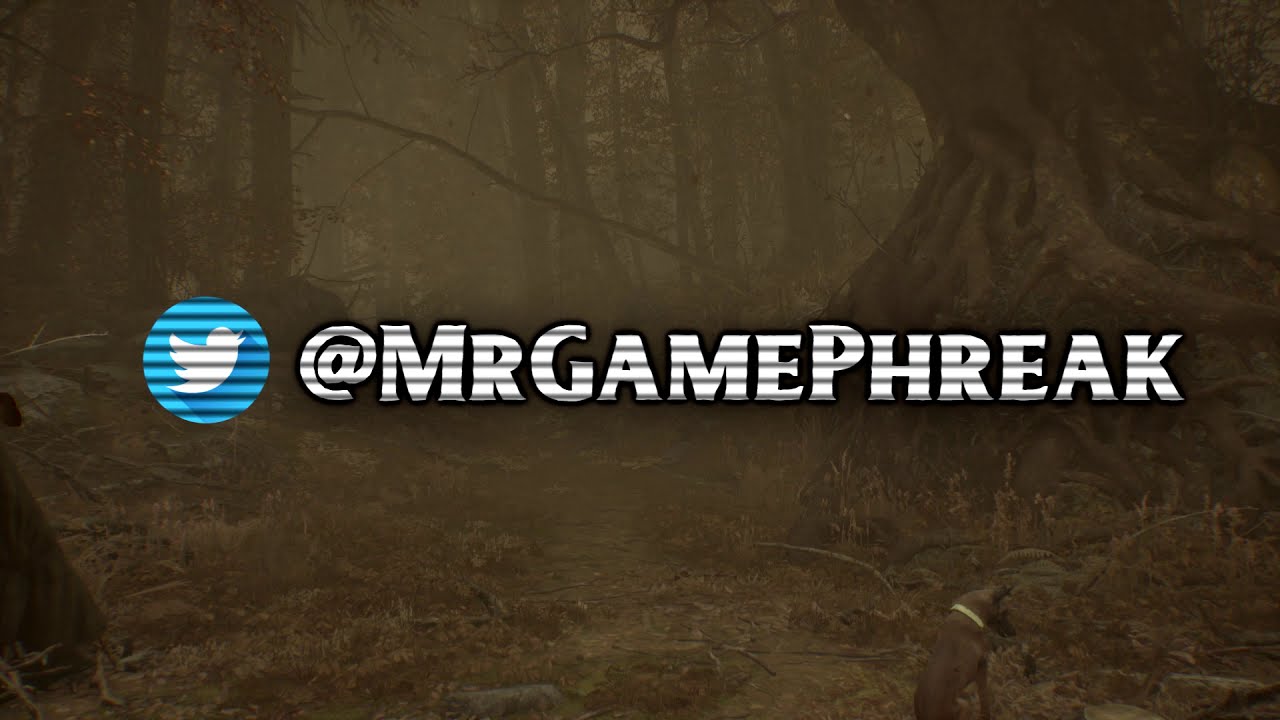The image is a heavily processed photo, giving it a painterly appearance, set in a dark woodland or forest scene. The background features various types of vegetation, including flowers and grass at the bottom. Multiple tree trunks are visible, with a large trunk on the right side and several others on the left, possibly framing a partial trail. In the upper right corner, a tree stump with extensive roots can be seen, stretching upward and to the left. Situated in the lower right corner is a dog wearing a light-colored collar, its back visible and head turned downward to the right. 

Prominently displayed in the middle of the picture is a Twitter logo with horizontal bars running through both the logo and accompanying text, creating a stylized "blinds" effect. The logo features a blue background with a white bird icon. Next to it, the Twitter handle "@MrGamePhreak" is written in white, capitalized text, with the letters "M," "G," and "P" significantly larger than the others. This text serves as an advertisement directing viewers to the user's Twitter page.